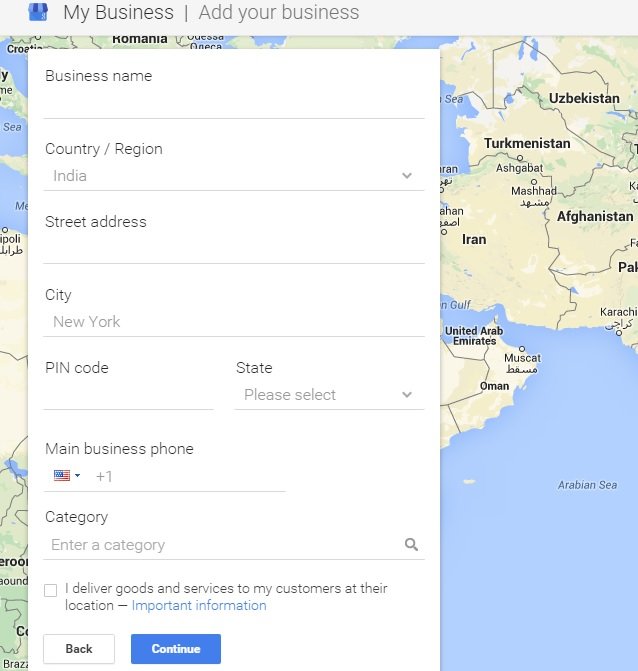The image showcases an online business directory interface. At the top of the screen, there are tabs labeled "My Business" and "Add Your Business." The background prominently features a detailed map that includes countries such as Romania, Iran, Turkmenistan, Afghanistan, Uzbekistan, and regions around the United Arab Emirates, all surrounded by bodies of water like the Arabian Sea.

Central to the image is a prominent listing form with a white background overlaying the map. The form is partially filled out: the "Country/Region" field contains "India," the "City" field is marked as "New York," and other fields like "Street Address" and "PIN Code" are currently blank. A drop-down menu prompts the user to select a state. Additionally, the form includes a section for a main business phone number, which features an American flag and a +1 country code indicating an American phone number.

The form invites users to enter a category for their business, with an hourglass icon situated at the far right of the entry line. Below this, a highlighted section provides guidance on delivering goods and services to customers at their locations. At the bottom of the form are navigation buttons, including a "Back" button and a prominently displayed bright blue "Continue" button.